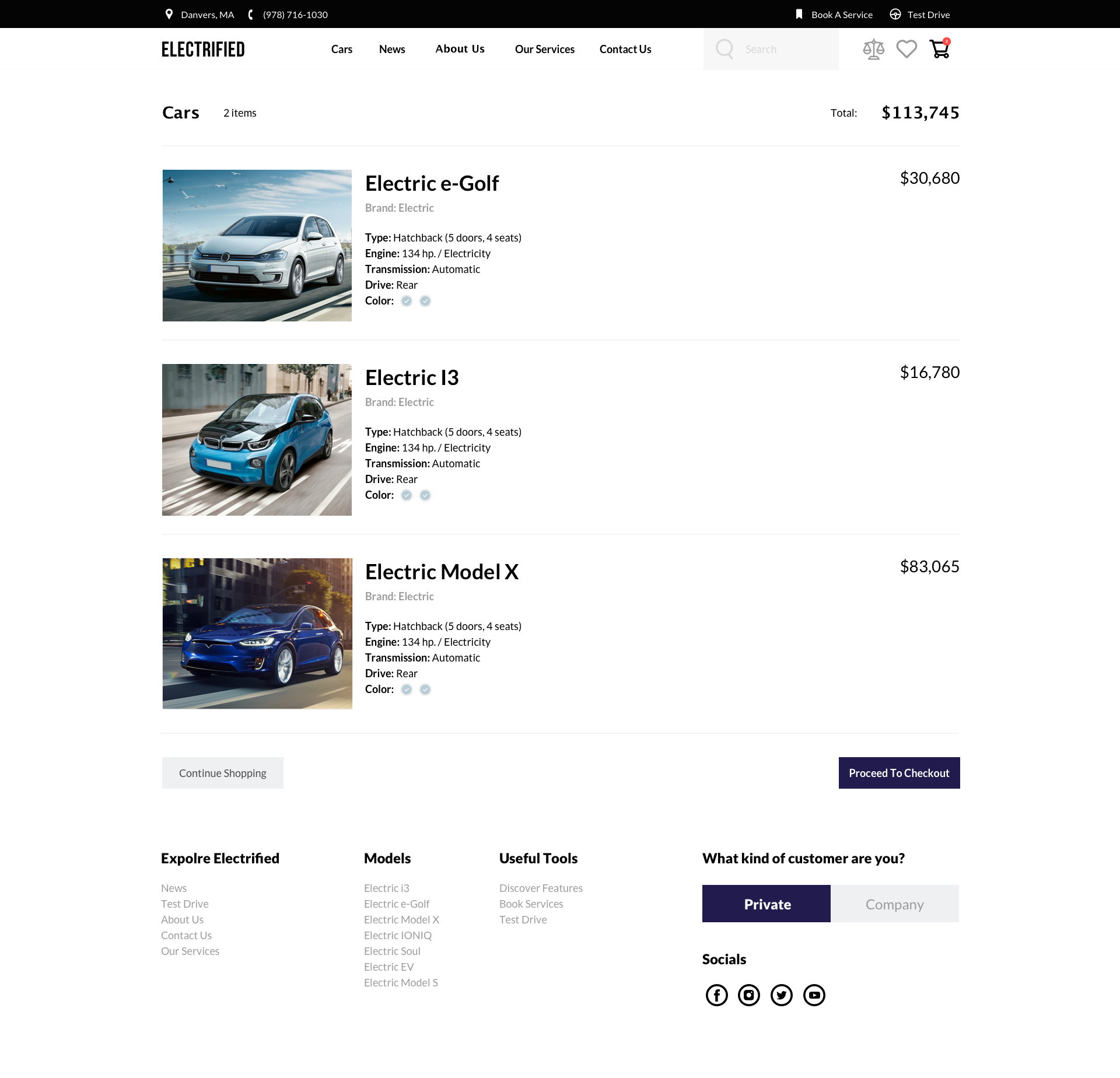In the image, there is a site header featuring a black rectangle at the top with words and symbols that are illegible due to their small size. Below it, the text "Electrified" is prominently displayed alongside navigation links: "Cars News," "About Us," "Our Services," and "Connection." To the right, there is a light gray rectangle hosting a magnifying glass icon, a scale symbol, an outlined gray heart, and a black shopping cart with a red dot, indicating potential interactive elements.

The body of the page contains various sections featuring electric vehicles, each accompanied by brief descriptions and price points. The first showcased car is labeled "Electric E-Golf," priced at $30,680, though the text underneath is too small to discern. Similarly, there are two blue dots below each vehicle description.

Further down, another vehicle titled "Electric 13" is displayed with an associated price of $16,780. This is followed by a section for "Electric Model X," priced at $83,065.

On the left-hand side, there is a vertical gray rectangle containing text that is unclear. Parallel to this is a purple rectangle on the right-hand side labeled "Explore Electrified," with an illegible description below it. Additional sections are labeled as "Models," "Useful Tools," and a segment titled "What Kind of Customer Are You?" with the options "Private" in a purple rectangle and "Company" in a gray rectangle. A footer section labeled "Socials" displays various social media icons, concluding the detailed layout of the image.